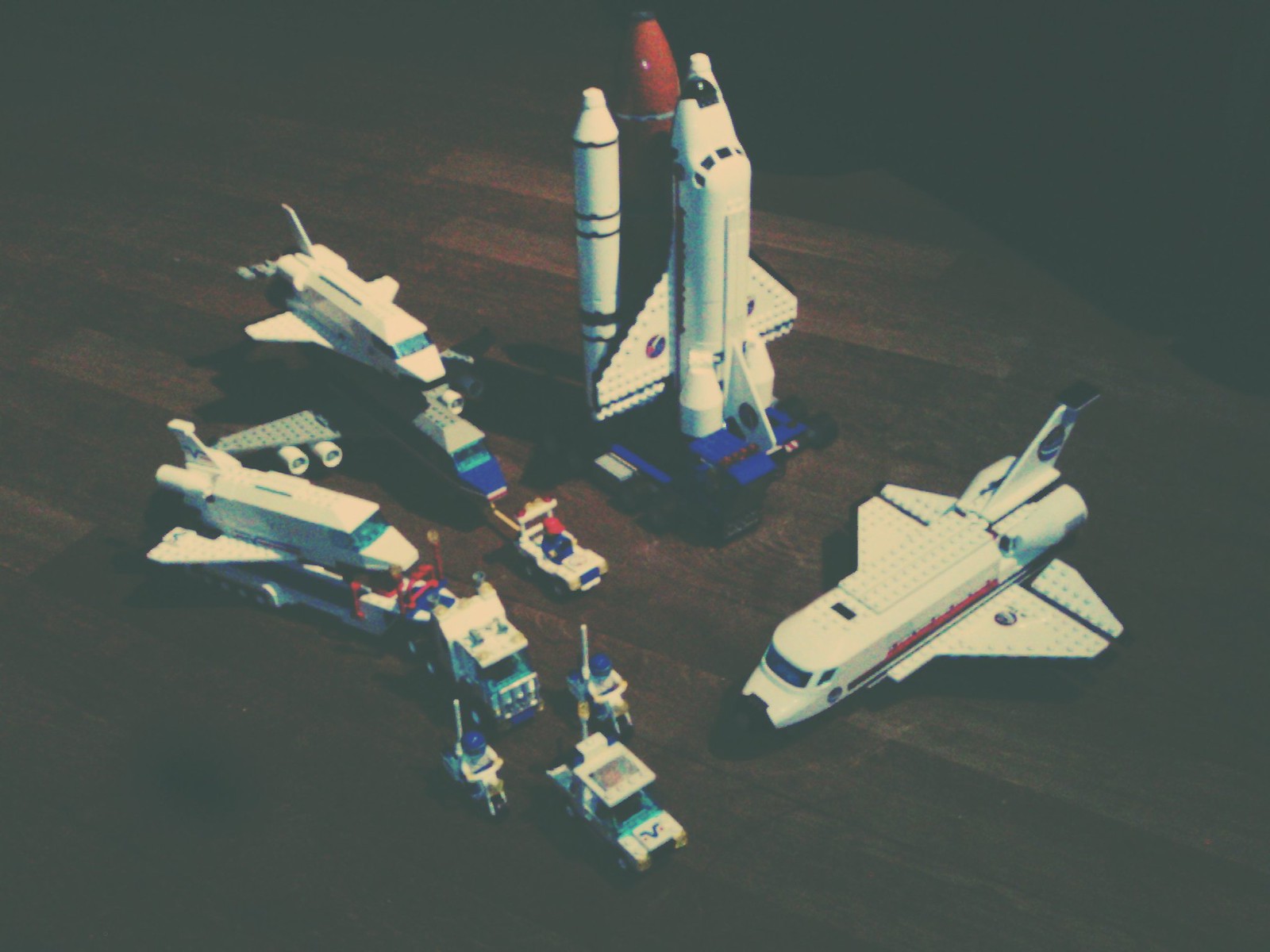The photograph captures an assembly of intricately built Lego models, all with a distinct space and NASA theme, displayed on a hardwood floor in dim lighting. Dominating the center of the image, a space shuttle equipped with three booster rockets stands vertically, poised for launch. To its right, another similar shuttle lies horizontally, seemingly at rest. Toward the top left corner, a smaller space shuttle can be seen. In the bottom left, a detailed convoy features a lead car, two motorcycles, and a semi-truck hauling an additional space shuttle mounted on its trailer. The models are predominantly white, with accents of blue and red, adding to their realistic, miniature space exploration aesthetic.